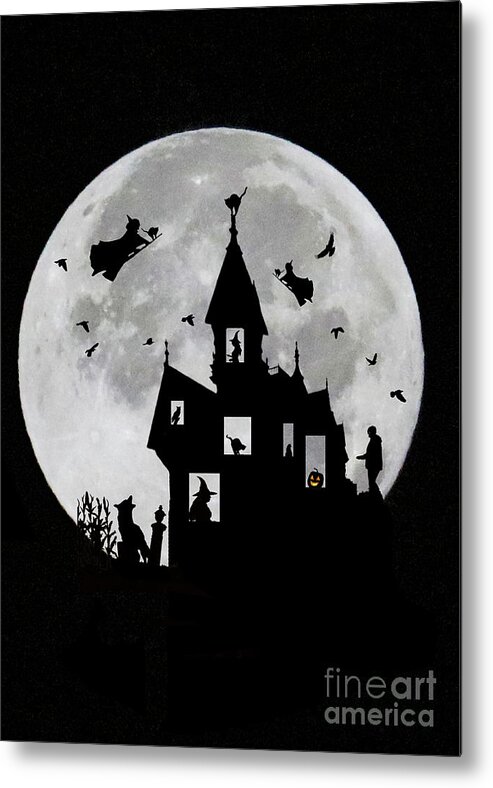This detailed canvas print from Fine Art America features a captivating Halloween-themed scene set against a black night sky with a full moon, whose surface reveals intricate craters. The moon acts as a backdrop to silhouettes of witches flying on broomsticks, accompanied by cats. Around them, crows are scattered, enhancing the eerie atmosphere. Centered in the image is an ominous, sharp-steepled haunted house with a distinct widow's peak, adding to its ghostly appearance. The windows of the house display various spooky elements including a jack-o'-lantern, silhouetted witches wearing pointed hats, and cats. On the ground near the house, an ambiguous figure, possibly a mummy or a man, is seen moving towards the front, with a dog or wolf lurking on the left-hand side.